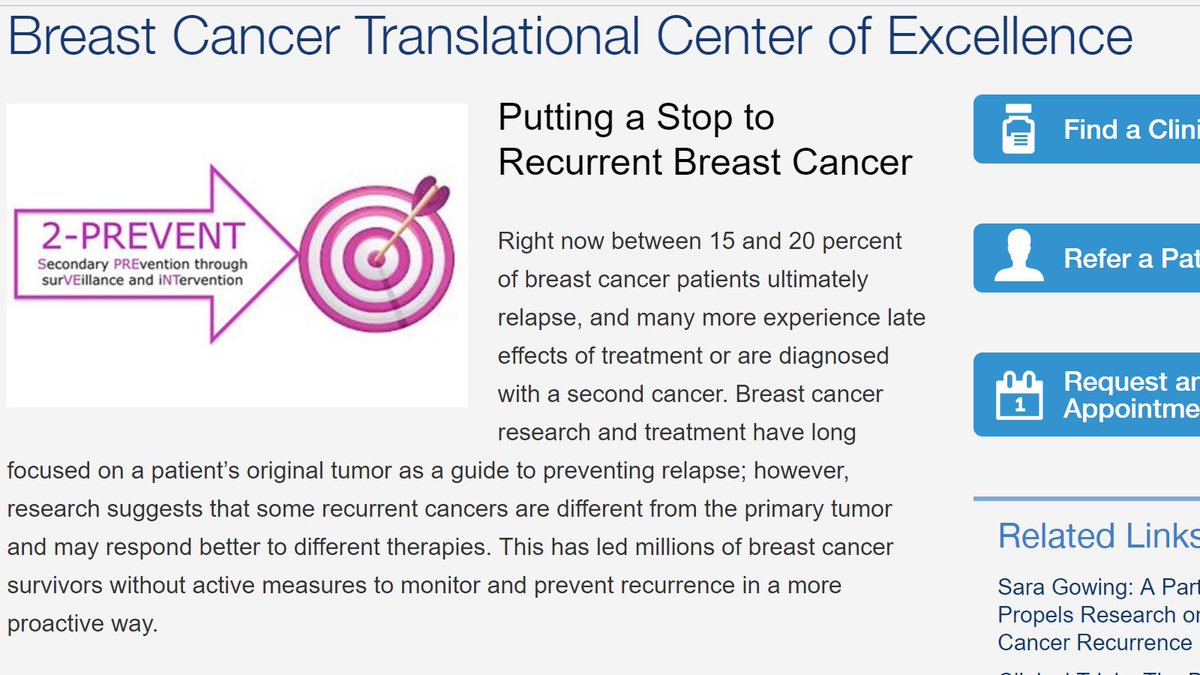The image is a screenshot taken from a website dedicated to breast cancer awareness, specifically the Breast Cancer Translational Center of Excellence. Dominating the top of the webpage is a large, prominent title that reads, "Breast Cancer Translational Center of Excellence: Putting a Stop to Recurrent Breast Cancer." Below the title, there is a significant paragraph conveying crucial information about breast cancer relapse statistics and the evolving approach in research and treatment. The text reveals that between 15 and 20 percent of breast cancer patients experience a relapse, with many others facing late effects of treatment or being diagnosed with a second cancer. Traditional breast cancer research has focused on a patient's original tumor to prevent relapse, but new studies indicate that some recurrent cancers differ from the primary tumor and may respond better to alternative therapies. Consequently, millions of survivors lack proactive measures to monitor and prevent recurrence more effectively.

The website features an all-white background, giving it a clean and clinical appearance. On the right-hand side, there are several blue buttons providing navigation options such as "Find a Clinic," "Refer a Patient," and "Request an Appointment." To the left and just below the main title, there is a graphic of a pink and white bullseye with an arrow hitting the center. Adjacent to this graphic, a caption reads, "To Prevent: Second Prevention Through Surveillance and Intervention."